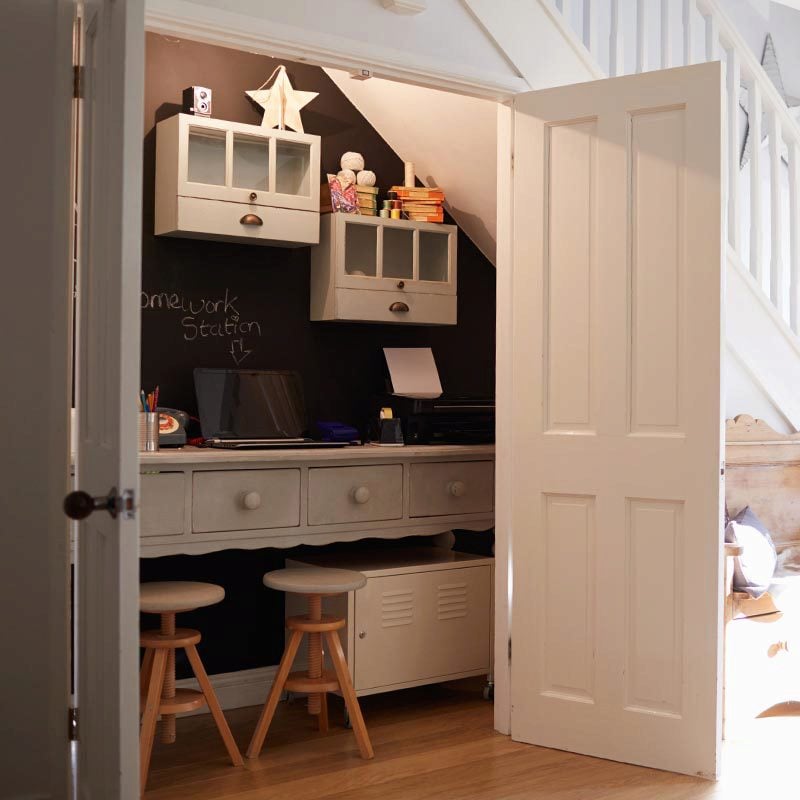This image is a full-color photograph taken indoors on a sunny day, showcasing a small, organized office space cleverly set up underneath a stairway. The vertically rectangular photograph has no border and conveys a bright atmosphere primarily colored in white. The focal point is a compact room accessible through a large set of white doors that swing out. The floor of this room and the surrounding area is hardwood.

Inside the office, there are two wooden stools with round white tops positioned under a built-in countertop. This countertop houses several white drawers, each with matching handles, further enhancing the tidy and minimalist aesthetic. Sitting on the countertop is a laptop, with a handwritten note in chalk behind it that reads "Homework Station," accompanied by an arrow pointing to the laptop screen. A silver can of pens or pencils is also placed on the counter.

On the wall above the countertop, there are two sets of white cabinets with glass-paned windows; one set is directly above the counter on the right, while the other is slightly to the left. These cabinets contain additional storage space and add an elegant touch to the small workspace. At the very top, a decorative star and what appears to be an old camera rest against the brown-toned background of the upper wall, where some boxes are also stored.

To the bottom right of the stools, there's a white locker-type cabinet with a key insert, adding another layer of functionality. In the background, the banister of the stairway is visible in the upper right, with sunlight filtering through a window, casting light onto the hardwood floor. A pillow can be seen in the lower right-hand corner, likely placed on a bench just out of the frame. Overall, this carefully staged photo captures a charming and practical home office nook, cleverly utilizing the space beneath a stairwell.